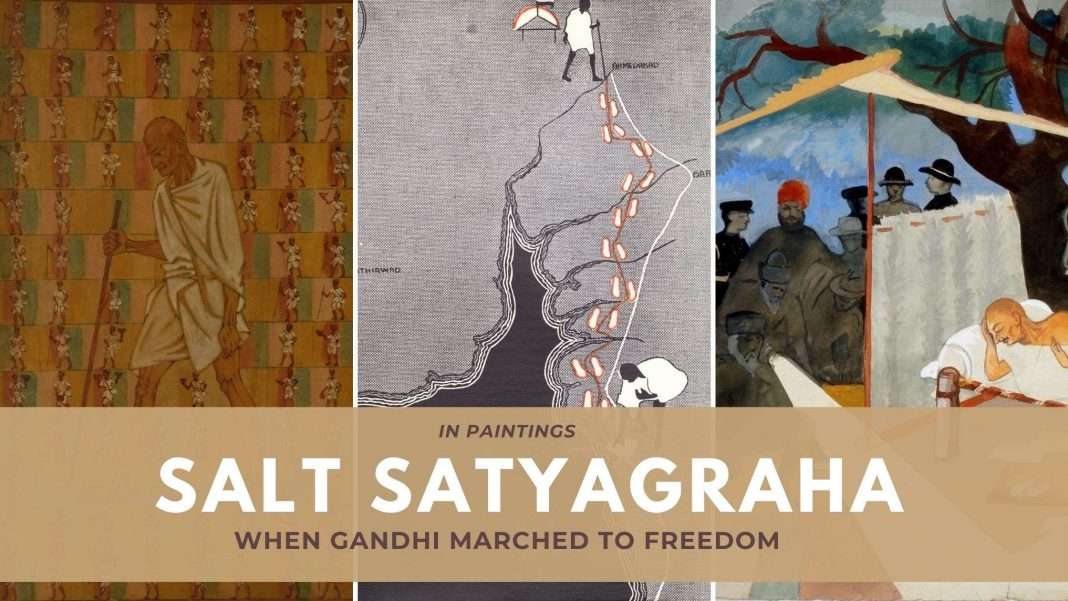The advertisement features a horizontal, wide rectangular image segmented into three vertical rectangles, each illustrating a scene related to Mahatma Gandhi. On the left, a painting portrays an older, brown-skinned man wearing a white robe and shorts, holding a brown wooden staff. This figure, representing Gandhi, walks with his head bowed amidst a patterned background of brown and green hues. The central image resembles a map in light and dark gray, depicting Gandhi’s march with a white line tracing his path. This section includes a black-and-white rendition of Gandhi as well. The rightmost painting showcases Gandhi lying in a white bed, potentially his deathbed, outdoors under a blue sky with a black tree nearby, surrounded by onlookers. A light brown horizontal banner stretches across the bottom of the artwork, with the text: "In Paintings, Salt Satyagraha" in bold white, followed by "When Gandhi Marched to Freedom" in black. The overall composition suggests an advertisement, possibly for an art gallery event, capturing key moments from Gandhi’s historic Salt March.